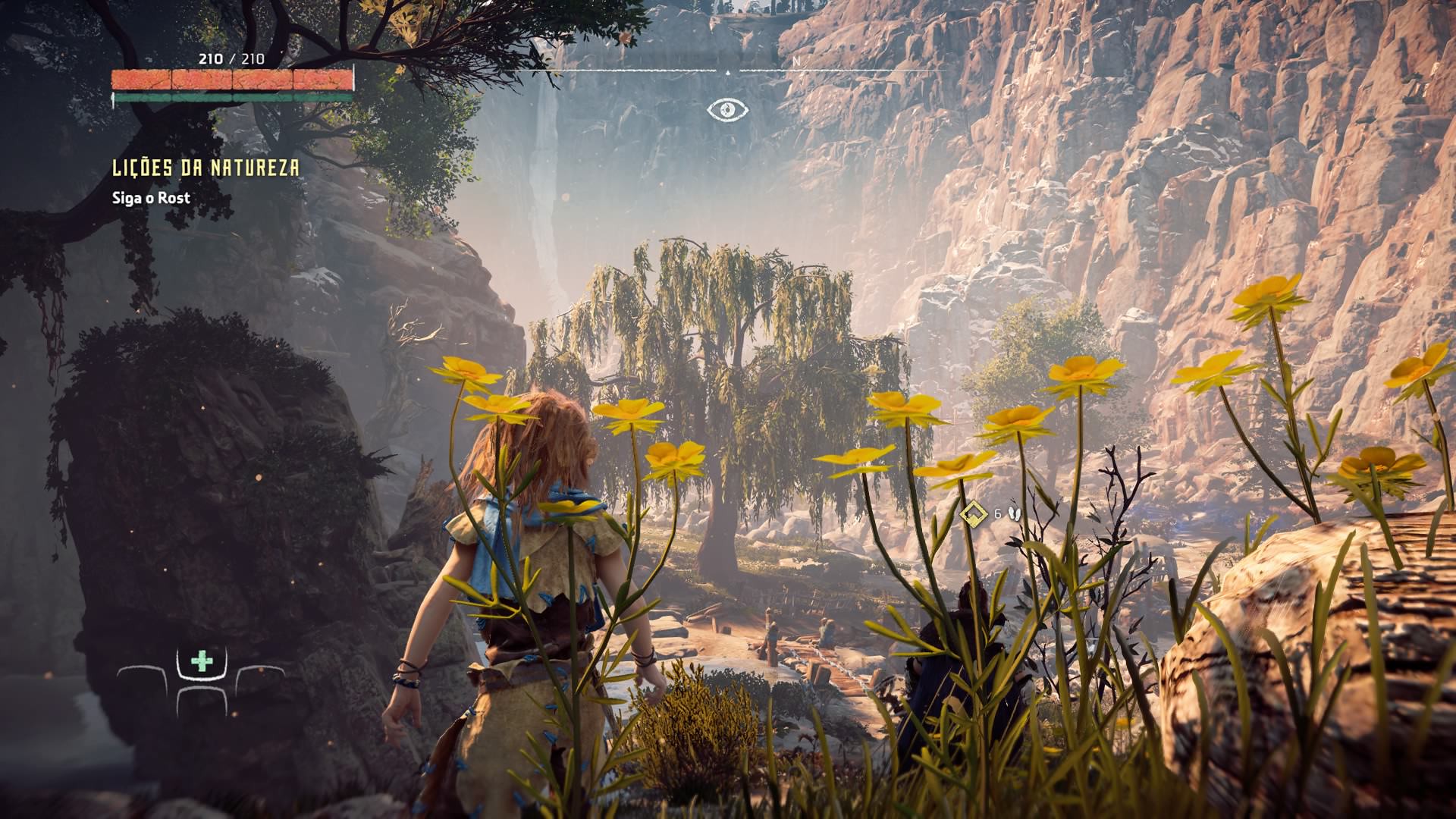A captivating nature scene unfurls in this image, capturing the rugged beauty of an arid landscape. To the right, a striking formation of tall, red rocks dominates the view, standing in stark contrast to the softer elements around them. On the left, the silhouette of a lone hiker adds a sense of adventure and human connection to the wild terrain. The hiker has long brown hair cascading down, and is clad in a khaki-colored outfit, complete with a sturdy backpack, indicative of a well-prepared explorer. She is navigating a winding nature trail, which meanders through the seemingly desert-like environment but remains vibrant with life. The sandy ground beneath her feet has a characteristic desert hue, though the presence of diverse plant life—including an assortment of trees, colorful flowers, and resilient shrubs—suggests a more complex ecosystem than a true desert. The overall scene marries the grandeur of red rock formations with the subtle, enduring beauty of desert flora, creating a picturesque and serene moment on the trail.